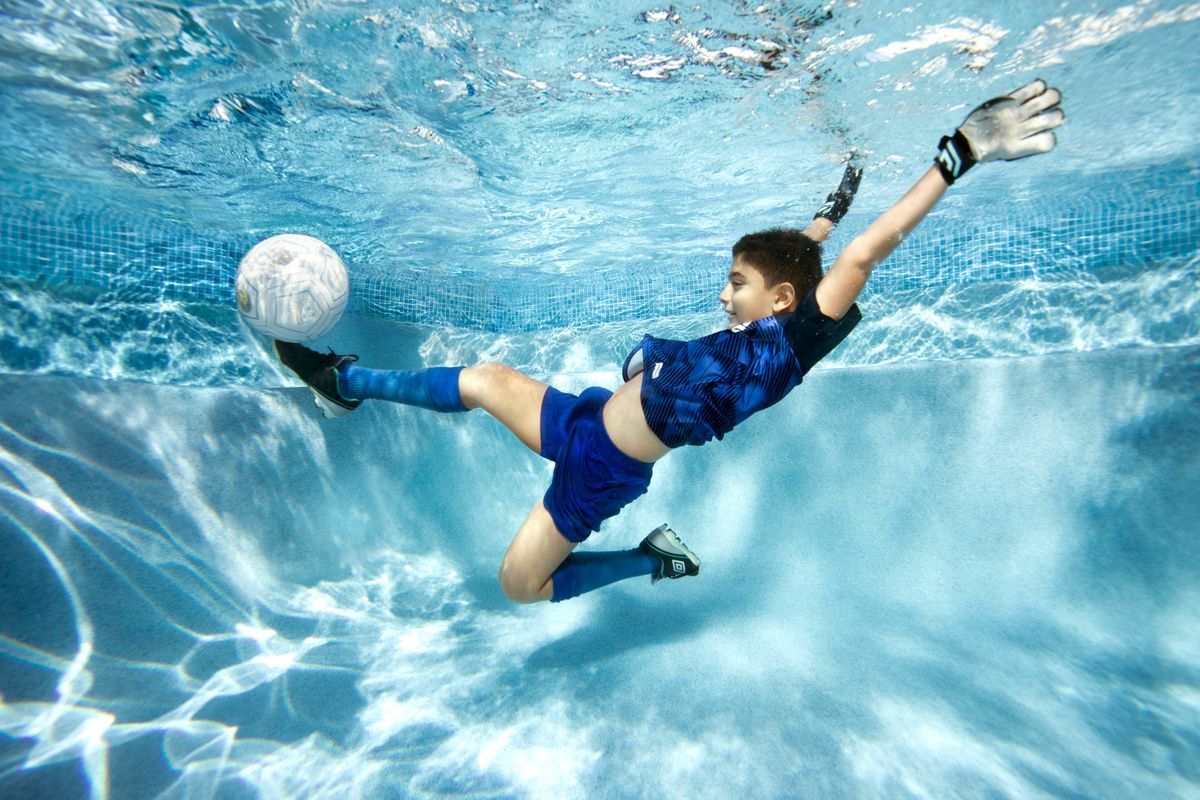This landscape-oriented color photograph captures an underwater scene of a young boy playing soccer in a swimming pool. The water is crystal clear with a light blue hue, revealing the pool's bottom surface, which is somewhat curved. The pool's sides feature a blue and light blue tiled checker pattern. The boy, positioned diagonally in the center of the frame, is fully kitted out in football gear, including a blue and black jersey, blue shorts, blue socks, white goalkeeper gloves, and dark football boots. His right leg is extended straight out as he kicks a white soccer ball, which is just touching his toe, while his other leg is bent under his body. His arms are stretched out toward the top right corner of the image, and his face is turned toward the left, focused intently on the ball. The photograph is a striking example of photographic representationalism and realism in underwater photography, capturing both the vibrant colors and dynamic motion of the scene. No text is present in the image.